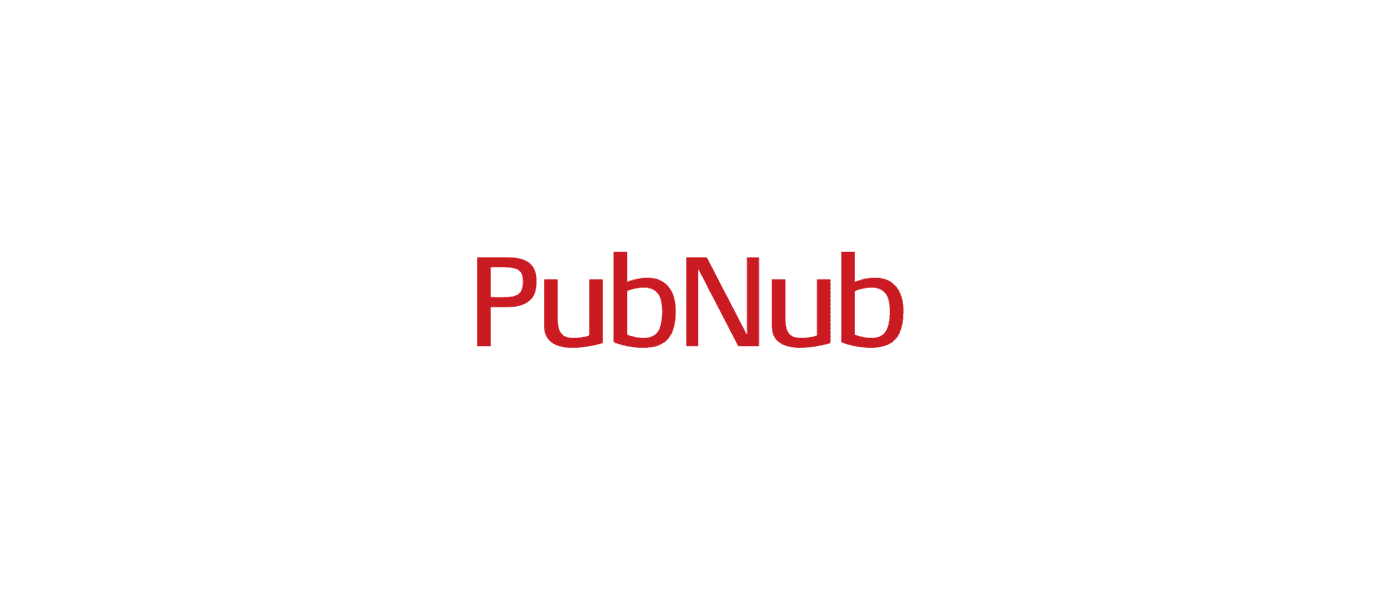The image features a central, horizontally aligned text on a plain white background. The text reads "PAP Nab" in bold red letters. The word "PAP" begins with a capital 'P', followed by lowercase 'a' and 'p'. The word "Nab" starts with a capital 'N' and is followed by lowercase 'a' and 'b'. The vibrant red text stands out sharply against the stark, unadorned white backdrop, drawing immediate attention to the wording in the center of the image. There are no additional elements or distractions—just the text "PAP Nab" prominently displayed.